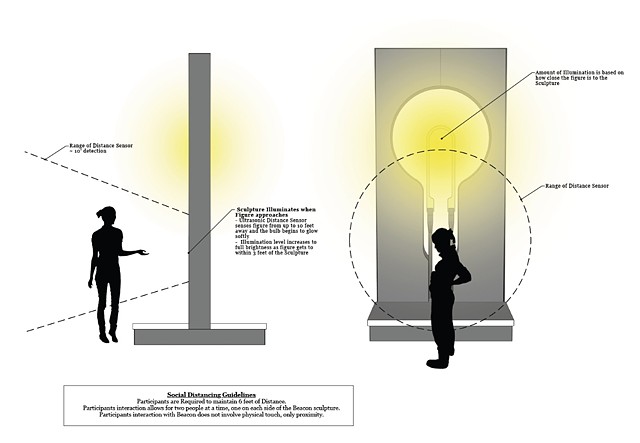This detailed diagram illustrates social distancing guidelines using black silhouette figures. Two clip art-style silhouettes, one of whom appears to be pregnant, stand facing each other on either side of an upside-down T-shaped beacon sculpture. The individuals, devoid of facial features, maintain a six-foot distance, following the guidelines displayed at the bottom of the image. The beacon, sensitive to proximity within a 10-foot range, illuminates as they approach without requiring physical touch. Detailed diagrams within the image highlight the correct distances required to activate the sculpture's yellow light, ensuring adherence to social distancing protocols.